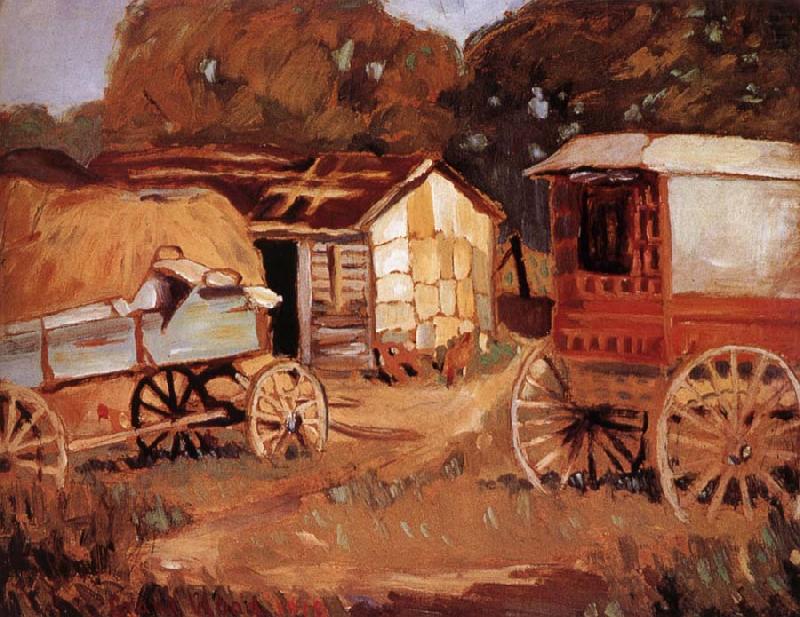This painting vividly captures a serene countryside scene dominated by warm, earthy tones of oranges, browns, and yellows. On the left side, there is a light brown stack of hay next to an open wagon with large, tall wheels. The hay gleams with golden hues, almost spilling out of the wagon. A wheelbarrow rests beside the haystack, adding to the rustic charm. On the right side, you see another prominent wagon, perhaps a covered carriage with its massive, light brown wheels and a reddish-orange body. This wagon, partially obscured by the front one, adds depth to the scene.

In the background, a rundown building stands with a patchwork appearance, as if constructed with mismatched wood. The roof, bearing etched lines, appears thatched and weathered, topped with a brownish, almost golden hue. Behind this aged structure, trees with orange-brown leaves rise, bathed in the gentle light of the setting or rising sun. At the bottom of the painting, sparse, greenish grass mingles with small bushes, grounding the composition and hinting at the seasons' changing.

The overall ambiance of this artwork exudes a nostalgic and tranquil countryside vibe, where the interplay of colors creates a harmonious and picturesque scene.